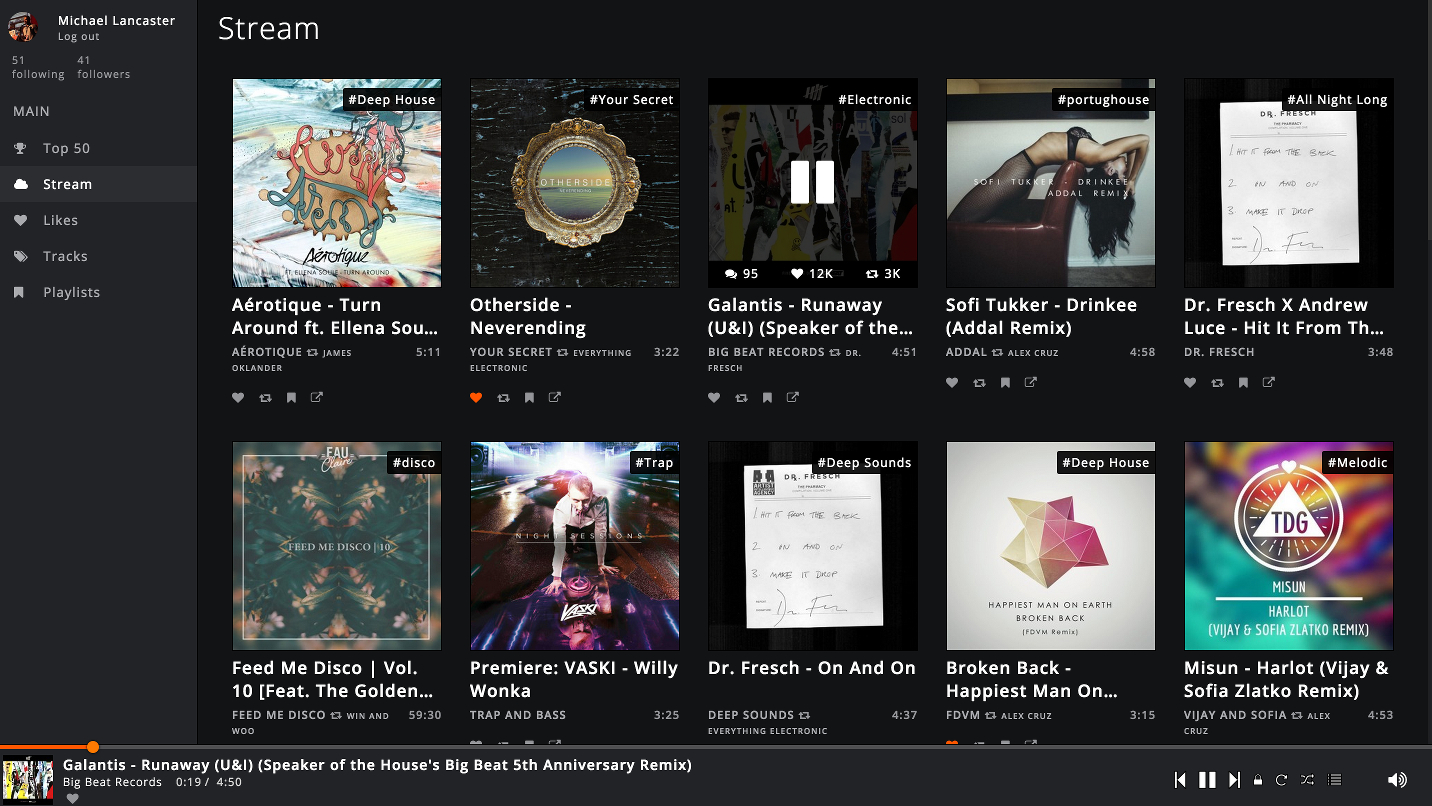In this screenshot of Michael Lancaster’s music streaming profile, a navigation menu is displayed vertically on the left, showing options like Main, Top 50, Stream, Likes, Tracks, and Playlists. Michael is currently viewing his "Stream" page, which features a grid layout with two rows, each containing five items.

In the first row, the top-left item displays an album cover for "AeroTique - Turn It Around" featuring Alina, followed by other titles like "Never Ending," "Your Secret," and "Everything." Next to it is Galantis' "Runaway (U & I)" with an additional note saying "Speaker of the..." The third item showcases Sofi Tukker’s remix of "Drinky." Lastly, Dr. Fresch's track "Hit It From The..." featuring Andrew Luce closes the first row.

In the second row, the first item is "Feed Me Disco Volume 10" featuring "The Golden..." continuing with a preview. Following that is "Premier Vaski - Willie Wonka" and another track by Dr. Fresch.

Overall, the profile reveals that Michael is following 51 accounts and has 41 followers.